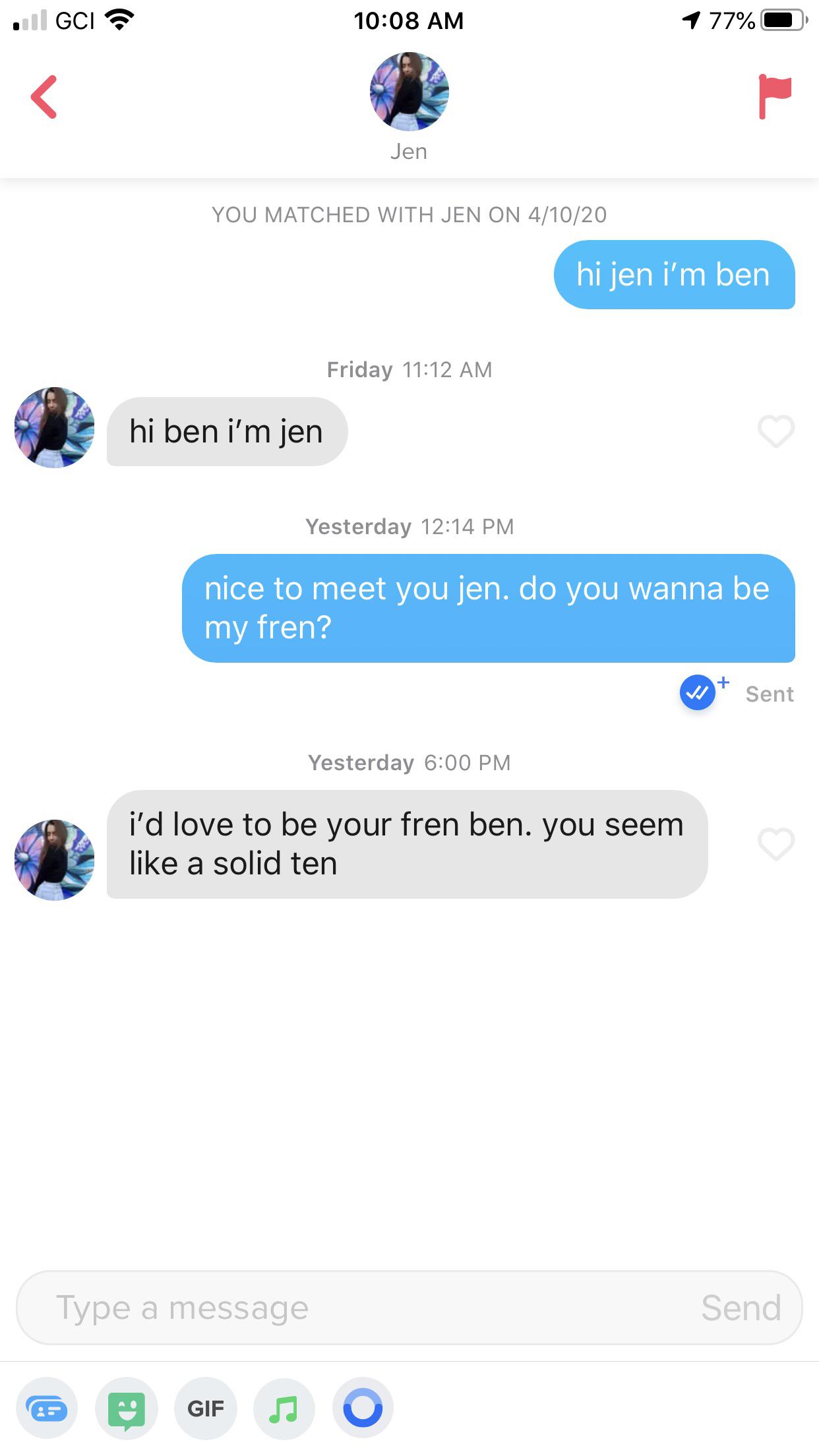**Screenshot of a Messaging Conversation**

In this detailed image, the screen captures a messaging conversation between two individuals. The interface background is white, typical of many modern messaging applications. 

**Top Section:**
- **Upper Left Corner:** Indicators for cell signal strength and Wi-Fi connectivity. The carrier is displayed as "GCI".
- **Center:** The current time is prominently displayed as "10:08 AM".
- **Upper Right Corner:** Icons for location services and battery status, with the battery at 77%.

**Mid-Section:**
- **Navigation and Profile:** 
  - A red back arrow for navigation is situated on the left.
  - In the center, there is a profile picture of a girl standing in front of a floral wall, labeled "Jin".
  - To the right, a red flag icon is present for reporting unwanted messages.

- **Subtext:** Indicates that the users matched on "4.10.20".

**Conversation:**
- **Ben:** "Hi Jin, I'm Ben."
- **Jin:** "Hi Ben, I'm Jin."
- **Ben:** "Nice to meet you, Jin. Do you want to be my friend? R-F-R-E-N to make it rhyme with Ben and Jin. Clever."
- **Jin:** "I'd love to be your friend, Ben. You seem like a solid 10."

This exchange showcases an initial introduction where the users playfully use rhymes to enhance their conversation.